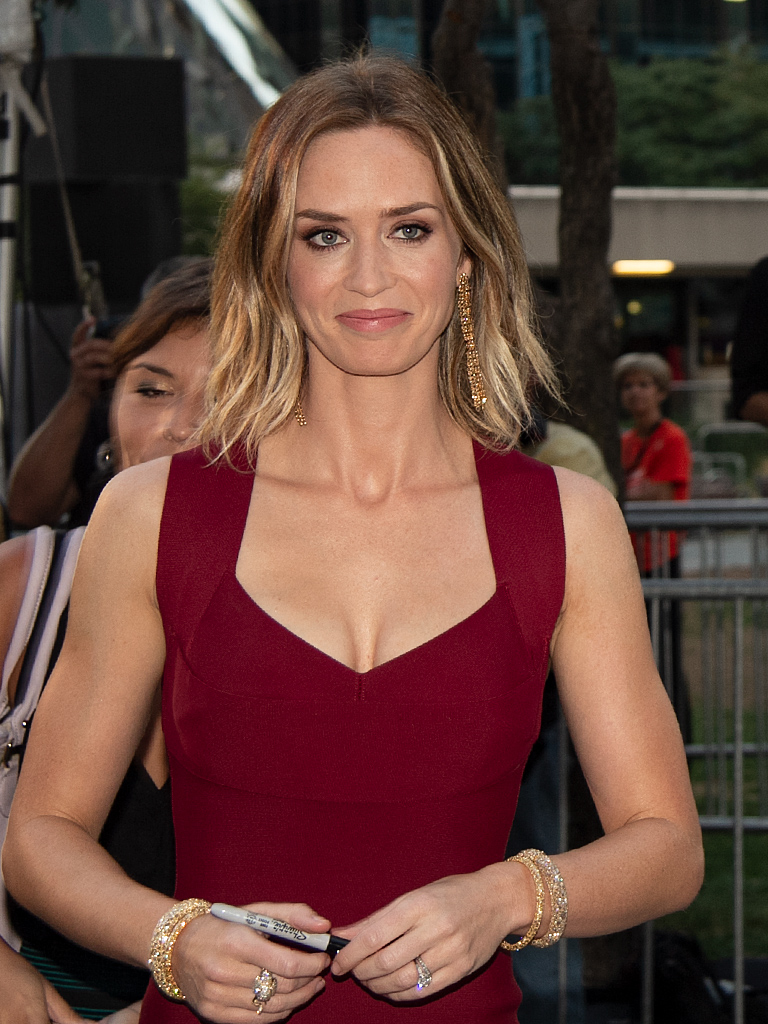The photograph captures a smiling actress in a fitted, maroon, halter-style dress with a low V cut, revealing a hint of cleavage. She has distinctive, shoulder-length blondish-brown hair with blonde streaks and is adorned with an array of gold and diamond jewelry, including long, dangling earrings, numerous bracelets on both wrists, and sparkling rings on both hands. She is holding a black Sharpie, suggesting she is about to sign autographs. Her makeup is meticulously done, with heavy eye makeup accentuating her strong cheekbones and bony facial features. The background shows a blurred crowd and a gate or fence, with several people behind her, indicating this is a public or event setting. She appears to be looking slightly off to the right, possibly at another camera.